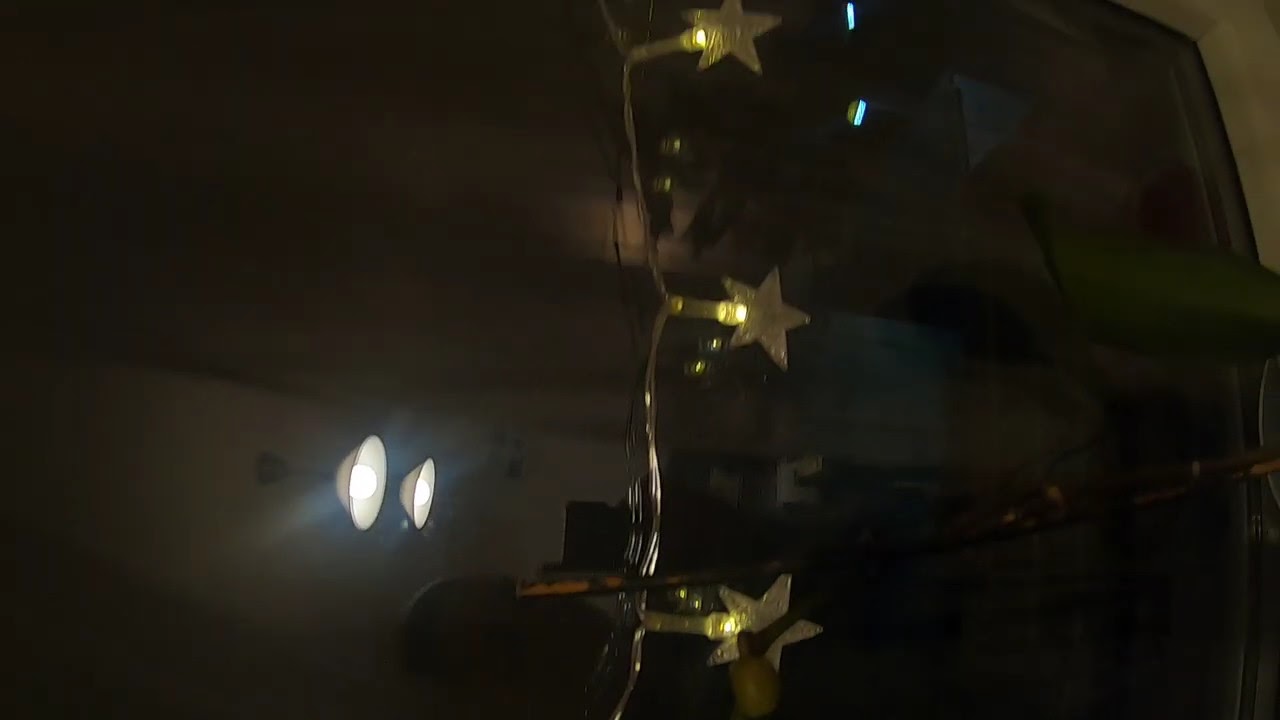The image, taken at night or in low lighting, is predominantly dark and somewhat blurry. Central to the scene are three golden-yellow, five-pointed stars, which hang vertically down the center of the photograph and occupy much of the space. These stars resemble decorations and are seemingly adorned with small white or LED lights, which are also gold-housed. The left side of the image features two incandescent bulbs with metallic shades, emitting a warm light that contrasts with the dark surroundings. The image might be a double exposure, adding complexity to its appearance. In the background, faint elements are visible - possibly a television and reflections of other light sources, or perhaps reflections on glass. The overall tone of the photograph ranges from brownish to very dark blue or black, further enhancing the difficulty in discerning finer details. The photo appears to have been rotated counterclockwise by 90 degrees, causing the ceiling lights to appear on the left side of the image.